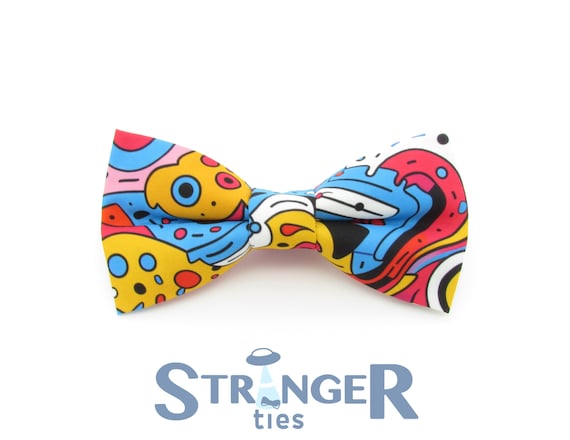The product photograph showcases a vibrant Dickie Bow style tie, centrally positioned against a stark white background. The tie's design is distinctly jazzy and abstract, featuring an array of bright, highly saturated colors including blue, pink, gold, white, black, red, orange, and yellow. Its pattern is intricate, comprising various shapes such as circles, rectangles, and stripes, evoking a pop art aesthetic. Below the tie, the text "Stranger Ties" is prominently displayed, appearing to be the brand's logo. The logo is distinctive, with the letter "A" stylized as a UFO beaming a bow tie, adding an imaginative touch to the design. The text is primarily blue, with the capital "S" and "R" being larger than the other letters. This product photo, ideal for an e-commerce website, captures the playful and eclectic essence of the tie, making it a standout accessory in fashion.